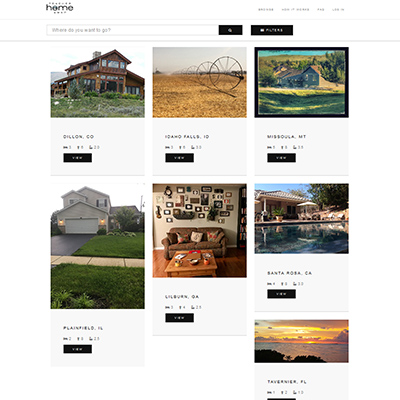The web page displays a neatly organized gallery of seven pictures arranged in three columns. In the first column, the top image showcases a large house with rustic wooden beams and walls, set on a lush grassy lawn. Below it, the second image presents a front view of a house, highlighting a garage door, green lawns, and a driveway. Moving to the second column, the uppermost picture captures a vast expanse of prairie land with dried brown grass and large wheels scattered across the scene. Below this, the second image in the column offers a cozy view of a living room furnished with a brown sofa, a wooden coffee table, and an array of framed pictures adorning the walls. The third column contains three more images, though their specific content is not detailed in the provided description. Each column effectively groups related visuals, enhancing the overall presentation of the web page.